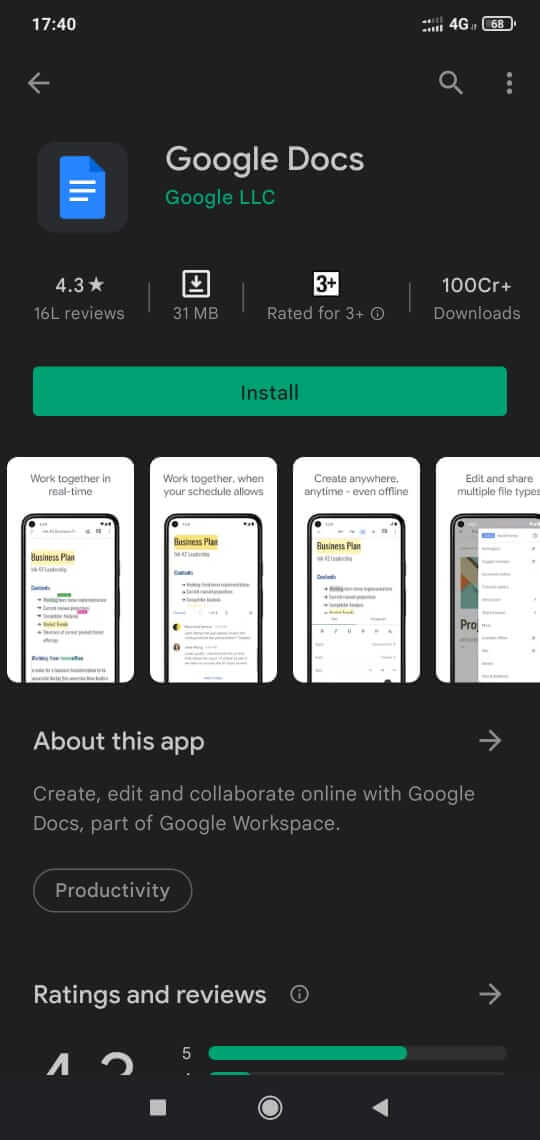A cell phone screenshot showcases the Google Docs app page on the Google Play Store. The background is black with the time "17:40" displayed in the top left corner, accompanied by the "4G" network indicator and a battery symbol on the right. 

In the middle of the screen, the app's name "Google Docs" is written in white text, with "Google LLC" in green beneath it. To the left, there is an icon of a blue sheet of paper with three horizontal white lines. The app has a rating of 4.3 stars, requires 31 MB of space, is rated for ages 3 and up, and has over 1,000 downloads. A green "Install" button is prominently featured.

Below, four informational sections appear, each depicting the app's interface on a cell phone screen with a white background and black text. The first section is titled "About this app" in white, followed by the description: "Create, edit, and collaborate online with Google Docs, part of Google Workspace."

Further down, the "Productivity" category is mentioned within a circular highlight. Beneath this, the "Ratings and reviews" section is marked with a small right-pointing arrow next to the rating "5." A green progress bar stretches almost to the right edge, indicating user satisfaction, with the remaining unfilled segment in black.